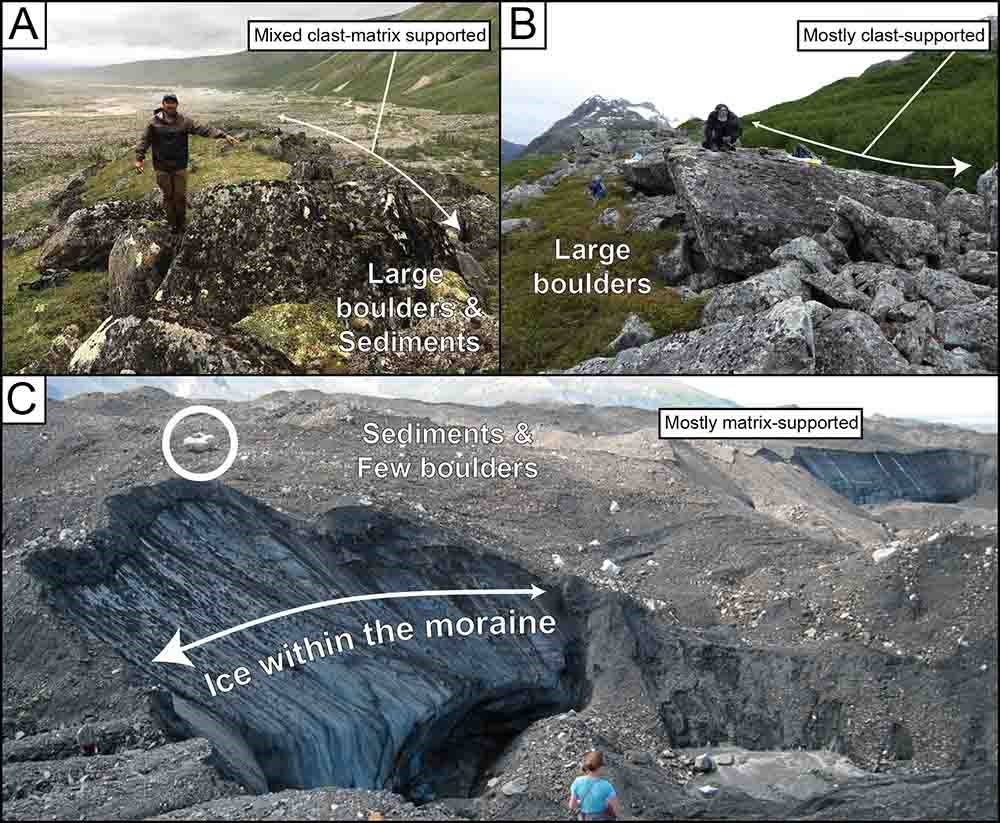The composite image consists of three differently labeled photos—A, B, and C—partitioned by black borders. Photo A, situated on the left, displays a rugged landscape with moss, grass, and large rocks in the foreground. Here, a man in a brown outfit and a baseball cap stands on a rock, pointing towards it. The scene is labeled "Mixed Clast Matrix Supported" and marked with white text indicating "Large Boulders and Sediments." In the background, a hazy sky and mountains add depth to the scene.

Photo B, located at the top right, captures a series of substantial, gray glacial boulders extending into the distance. A man, dressed in black, sits atop one of these boulders, appearing to work on something, while another person is visible hiking beside the boulder line. This image, labeled "Large Boulders, Mostly Clast Supported," features greenery and snowy peaks in the background, suggesting a colder climate.

Photo C, which spans the bottom half of the composite, showcases a sandy excavation-like landscape dotted with smaller rocks and striking blue ice flows within the moraine. This image is titled "Sediments and Few Boulders," with an arrow indicating "Ice Within the Moraine," and marked as "Mostly Matrix Supported." A woman in a light blue shirt observes the scene, which contrasts sharply with the surrounding gray rocks.

Collectively, these photos, set in diverse mountainous terrains, highlight different geological formations and the interplay between large boulders, sediment, and ice.